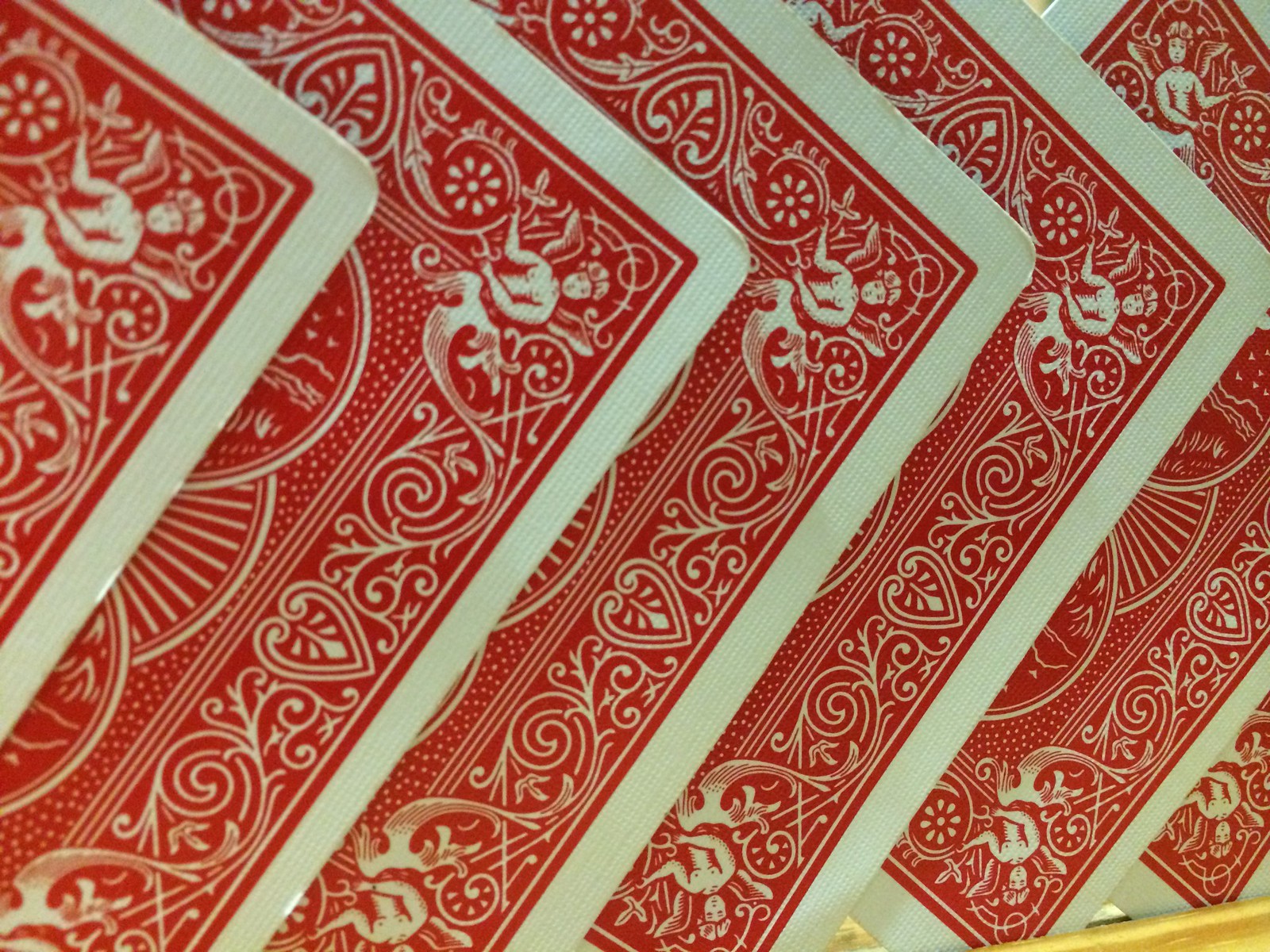The image depicts six red Bicycle playing cards arranged in a slightly fanned-out manner, showcasing their intricately designed backs. Each card features a white border and is adorned with detailed artwork, including an elegant figure, possibly an angel or a woman with a long tail, surrounded by various decorative elements. The cards obscure their denominations, focusing exclusively on the ornate patterns on the reverse side. In the background, a small portion of a brown drawer, slightly ajar, can be seen, with a white handle peeking out. A slender crack between the cards hints at the underlying surface, adding depth to the composition.